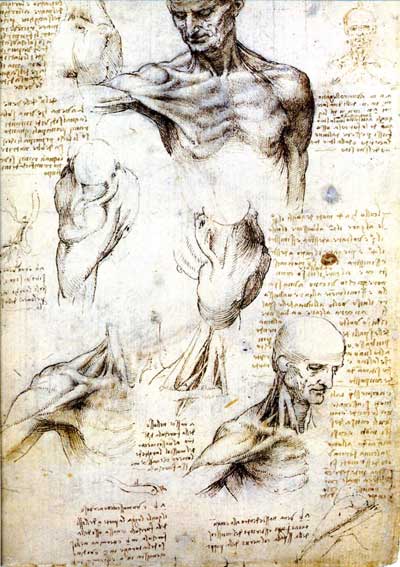This image features an aged and weathered illustration page, meticulously created in pencil. At the center and edge of the composition is an older man, depicted in various anatomical perspectives reminiscent of historic medical or artistic studies. The top section showcases a detailed view of his face and chest, revealing the structure of his muscles. To the left, his shoulder is intricately drawn, while at the bottom, the man is seen looking downward, providing a different angle of his musculature. Surrounding these illustrations is a wealth of handwritten notes in light brown ink, adding a scholarly touch to the artwork. The page itself is yellowed with time, showing a gradient from a more whitish center to deeply splotched grey and yellow edges, along with an assortment of textured markings indicative of its age and historical significance.